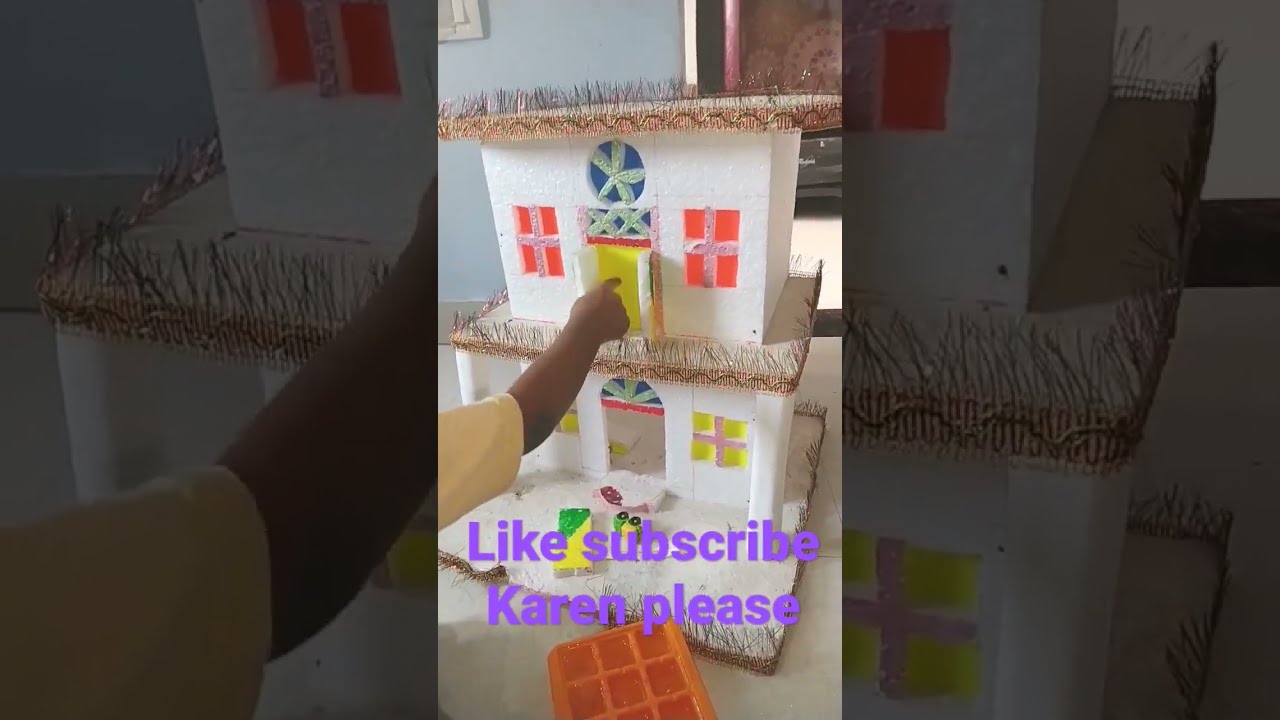The image is a color photograph in portrait orientation, centered with a darkened, landscape-oriented background that is an enlarged portion of the same photograph, likely formatted for a social media post. The focal point is a detailed, two-story white dollhouse sitting on a brown base with white paint. It features a brown roof with gold thatch grass-like edging. The structure has colorful windows: orange windows on the top floor, and yellow windows on the bottom floor. The top floor also includes a round blue window with a white star pattern and a doorway with a yellow background. The bottom floor has an arched entrance. A black arm is opening the door or a window, pointing towards the second floor. In the foreground of the image, there are the words "Like, Subscribe, Karen, Please" in lavender purple lettering, indicating a video, freeze-frame style typical for social media.